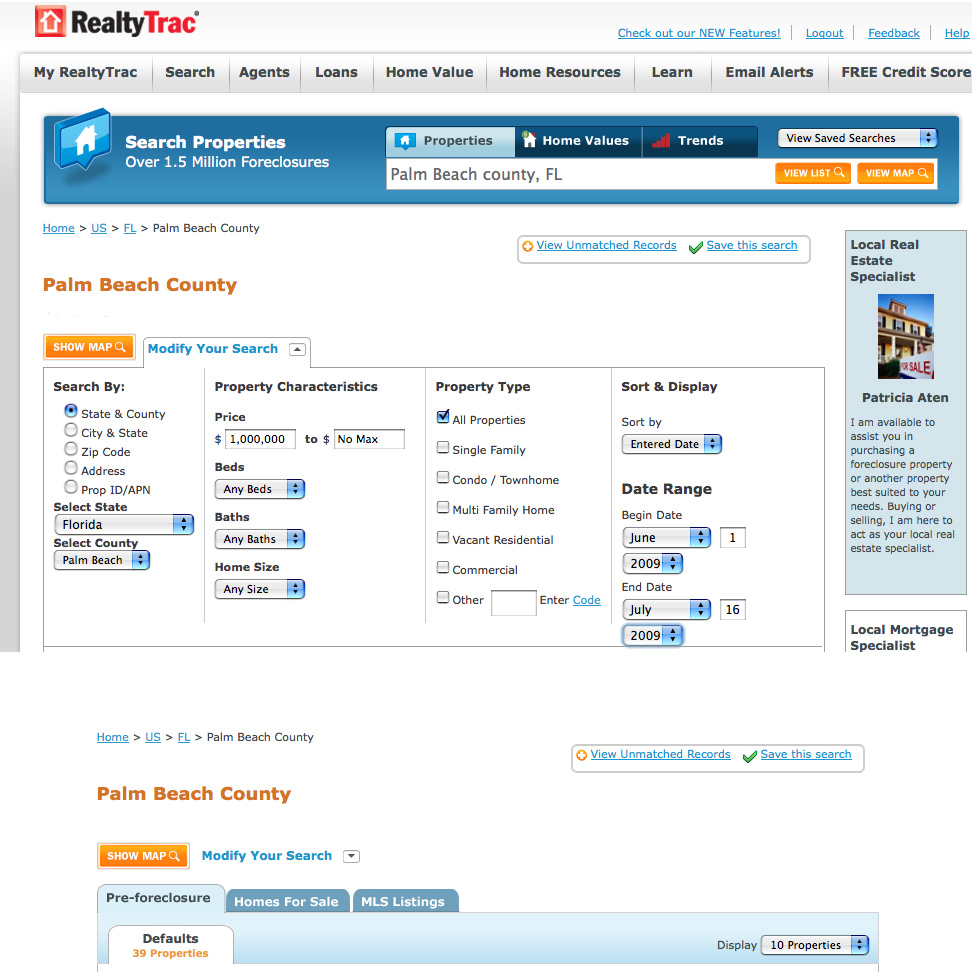This screenshot depicts a web page from the RealtyTrac website, identifiable by its logo, which features a white house icon inside a red square. The website's name "RealtyTrac" is displayed next to the logo, with several tabs positioned to the right: "Check Out Our New Features," "Log Out," "Feedback," and "Help."

Beneath this header, an additional row of navigation tabs includes options such as "My RealtyTrac," "Search," "Agents," "Loans," "Home Value," "Home Resources," "Learn," "Email Alerts," and "Free Credit Score." Just below, a prominent advertisement encourages users to search properties, boasting a database of over 1.5 million foreclosure listings.

The search interface itself offers multiple filtering options and functionalities. Tabs for "Properties," "Home Values," and "Trends" sit above a section where users can view and save searches. The default search location is set to Palm Beach County, Florida, with options to view results by list or map.

A navigation path is displayed ("Home > U.S. > Florida > Palm Beach County") along with options to view unmatched records and save the search. Users have the ability to show a map or modify their search criteria, which can include state and county, property characteristics (such as price, bed/bath count, home sales, home size, and property type). Types of properties include all properties, single-family homes, condos/townhomes, multifamily homes, vacant residences, and commercial properties. Users can also enter a specific code or sort and display results by various date ranges.

To the right, an advertisement promotes Patricia Atten as a local real estate specialist, alongside a local mortgage specialist. The current search results page continues to focus on Palm Beach County, highlighting tabs for "Preforeclosure Homes," "Homes for Sale," and "MLS Listings," with a display note indicating 10 properties out of the total 39 defaults being shown.